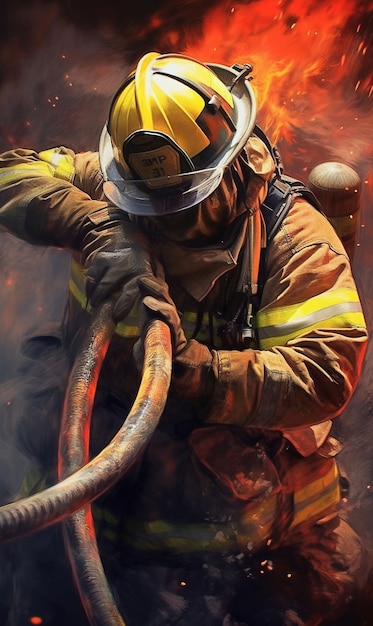This painting portrays a resolute firefighter in the midst of battling a fierce blaze. Clad in a yellow helmet and a tan fire-retardant coat with yellow and silver stripes, the firefighter's face is obscured, likely by protective gear against the thick smoke billowing around him. He holds a hose, gripping it firmly with gloved hands, as he pulls it towards the flames that rage in the background. The bright orange fire turns black at the edges, hinting at the intense heat and chaos. Despite the inferno, the firefighter remains focused on his duty to extinguish the fire and ensure everyone's safety. His posture and the visible oxygen tank on his back underscore his determination and readiness to save lives, embodying bravery and resilience. The close-up view accentuates the urgency and gravity of the scene, making the viewer almost feel the heat and tension depicted.